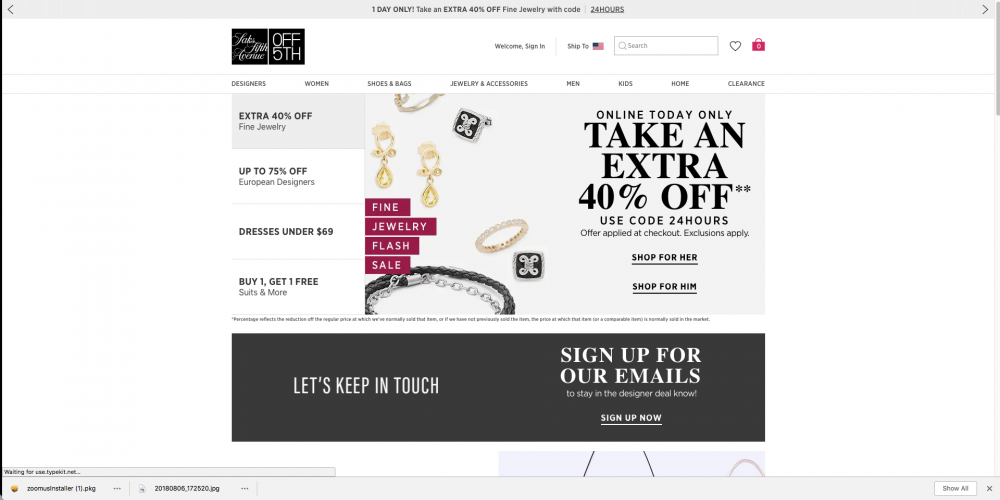Here is a refined and detailed caption for the described image:

---

This promotional image showcases an exclusive "One Day Only" sale from the Saks Fifth Avenue OFF 5TH website. The image's layout includes distinctive borders and text sections, contributing to an organized and eye-catching design.

- **Top Section**: A light gray strip, about a quarter inch thick, spans the top of the image, contrasted with bold black text that reads "ONE DAY ONLY! TAKE AN EXTRA 40% OFF". This header immediately captures attention.

- **Borders**: The left side of the image is edged by a thin black line, while the right side features a slightly lighter gray line. The bottom of the image has a half-inch gray border, grounding the overall design.

- **Header Content**: Positioned toward the top left, within a black square, the "Saks Fifth Avenue" logo is prominently displayed in white text. Adjacent to this, another black square contains the "OFF 5TH" logo, also in white. Midway across the top, there is the text "Welcome, Sign In," followed by a "Ship To" notice accompanied by an American flag icon. Further right, a gray search bar, a heart icon with a black outline, and a red bag icon are displayed.

- **Navigation Bar**: Below the header, a navigation menu in black text on a white background lists categories from left to right: Designers, Women, Shoes & Bags, Jewelry & Accessories, Men, Kids, Home, and Clearance.

- **Sale Announcement**: A gray rectangle on the left announces "EXTRA 40% OFF", linking to additional sale details. To the right, the primary promotional message is highlighted in a large, white-centered square with bold black text: "ONLINE TODAY ONLY. TAKE AN EXTRA 40% OFF. USE CODE 24HOURS".

- **Jewelry Preview**: The left side of the main section features images of various jewelry pieces, enhancing the visual appeal and relevance to the sale.

- **Flash Sale Information**: Midway down on the left, red rectangles with white text sequentially highlight key sale terms: "FIND", "JEWELRY", "FLASH", and "SALE".

- **Footer**: Spanning the bottom is a black rectangle with dual white texts. On the left, "Let's Keep In Touch" invites customer engagement, while on the right, "Sign Up For Our Emails" encourages newsletter subscriptions, accompanied by smaller text in white, "to stay in the designer deal know." Below it, "Sign Up Now" is underlined for emphasis.

---

This detailed description provides a clear visual representation of the promotional image, emphasizing the key elements and layout.